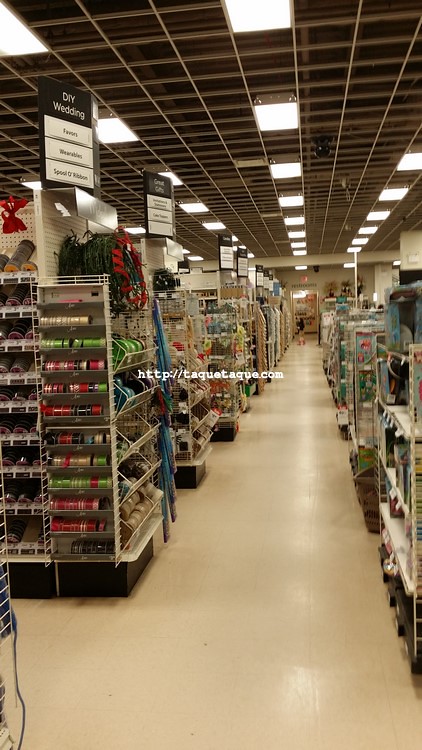The image showcases the interior of an arts and crafts store, providing a detailed glimpse into its layout and offerings. In the center of the photograph is a clean, white-tiled walkway that guides customers through the store. On the left side of the walkway, various aisles run perpendicularly, each marked with signs indicating different product categories. The front aisles prominently feature a white rack displaying a colorful array of ribbons. Each aisle is lined with multiple racks holding various crafting supplies. On the right side of the walkway, there are crates filled with merchandise, including a selection of toys. One of the toys, a doll, is noticeably packaged in a rectangular box. The store's ceiling is fitted with numerous square lights, brightly illuminating the space. Additionally, a black surveillance camera is mounted above, ensuring store security.